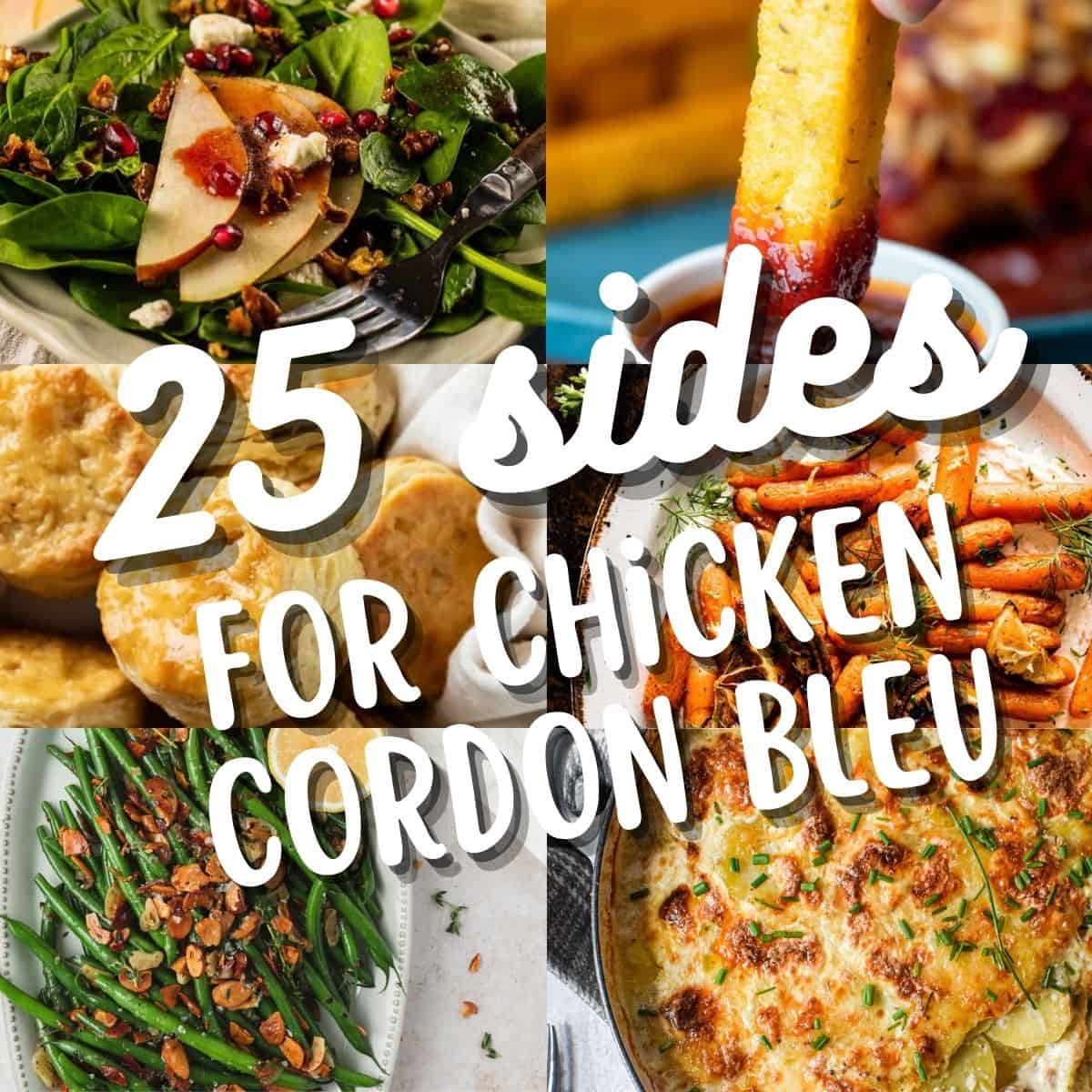The image is a detailed advertisement or Pinterest-style thumbnail showcasing a variety of side dishes that complement chicken cordon bleu, with the prominent text "25 Sides for Chicken Cordon Bleu" in large, white font centered for clarity and emphasis. The poster features six equally sized food images arranged in two vertical columns. The top left image exhibits a vibrant salad, possibly adorned with apples, leafy greens, and bits that could be bacon or raisins. Adjacent to it on the top right, a crispy french fry is being dipped into a bowl of ketchup. The middle row presents freshly baked, fluffy biscuits on the left, while the right side features herb-topped roasted carrots. For the bottom row, the left image shows a platter of roasted green beans, and the bottom right likely displays a cheesy potato dish. Each image collectively illustrates a variety of flavorful and visually appealing side options to pair with chicken cordon bleu.